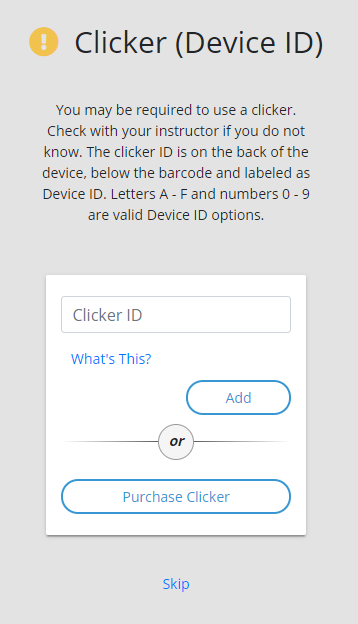The image is a vertical screenshot, likely captured from a smart device such as a smartphone, tablet, or computer. The background is a uniform medium gray color without any texture or dimension. At the top of the image, there is an orange circle containing a light gray exclamation point, indicating important information.

To the right of the orange circle, in black text, the word "Clicker" is displayed, followed by "Device ID" in parentheses. Beneath this, in smaller black font, a detailed instruction reads: "You may be required to use a clicker. Check with your instructor if you do not know. The clicker ID is on the back of the device below the barcode and labeled as device ID. Letters A through F and numbers 0 through 9 are valid device ID options."

Below this text, a white rectangular box is positioned prominently against the gray background. Inside this box, there is a field labeled "Clicker ID," with a blue link labeled "What's this?" directly underneath. Next to the "Clicker ID" field is an "Add" button. Further down, a circle encloses the word "or," providing an alternative option.

At the bottom of the white box, a button labeled "Purchase Clicker" is available for users. Finally, at the very bottom of the image, a blue "Skip" link offers an option to bypass the current interface.